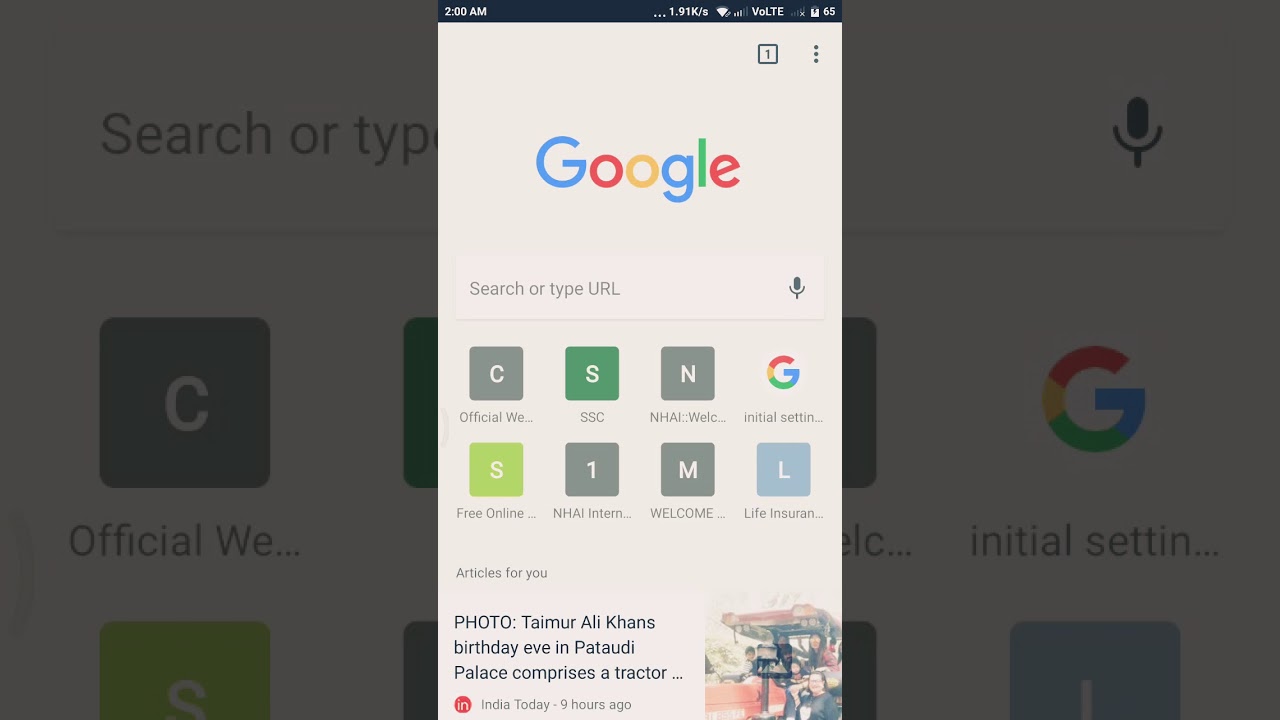In the center of the image, there is a prominent vertical and rectangular-shaped pop-up that appears to be a Google app interface. At the top left of this pop-up, the current time is displayed as 2 AM. Dominating the middle section is the word "Google," with each letter distinctly colored – the 'G' in blue, the first 'o' in red, the second 'o' in yellow, the 'g' in blue, the 'l' in green, and the 'e' in red.

Directly below the Google logo, a rectangular search bar invites users to "search or type URL." Positioned at the far right of the search bar is a small microphone icon, indicating the option for voice search.

Beneath the search bar, there are eight square icons representing frequently visited websites. The icons are arranged in two rows of four. The first row includes icons labeled 'C', 'S', and 'N', followed by an icon with the Google logo. The second row features icons labeled 'S', '1', 'M', and 'L'.

Further down, the section titled "Articles for you" presents personalized content. The first article headline reads: "Photo: Timer Ali Khan's birthday eve in Padoody Palace compromises a tractor." To the right of this article's headline is an image depicting a group of people.